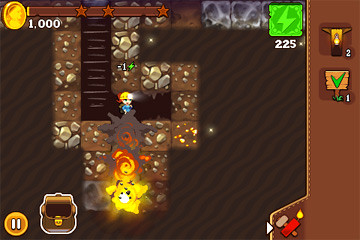This image is a low-resolution screenshot from a mobile or video game featuring a digging or mining theme. The game’s environment is predominantly brown, resembling dirt, through which a character equipped with a hard hat is drilling. The backdrop of the game grid is interspersed with rock squares, indicative of the mining activity. The character appears to have cleared a path, potentially using an explosive, as evidenced by an ongoing explosion in the scene.

In the game's user interface (UI) at the top left, there is a golden coin-like avatar. To its right, a brown progress bar extends, marked with three stars and displaying the number 1,000 underneath. Adjacent to this is a green square with an electrical symbol, alongside the number 225. On the right side of the screen, an in-game menu or inventory is visible with icons displaying quantities; notably, one icon shows ‘2’ and another signpost icon shows ‘1’. The menu area is bordered with stitching-like designs.

At the bottom left corner, there's an icon of an open brown satchel with a golden clasp, accompanied by a circular button featuring a pause symbol positioned in the bottommost left corner.